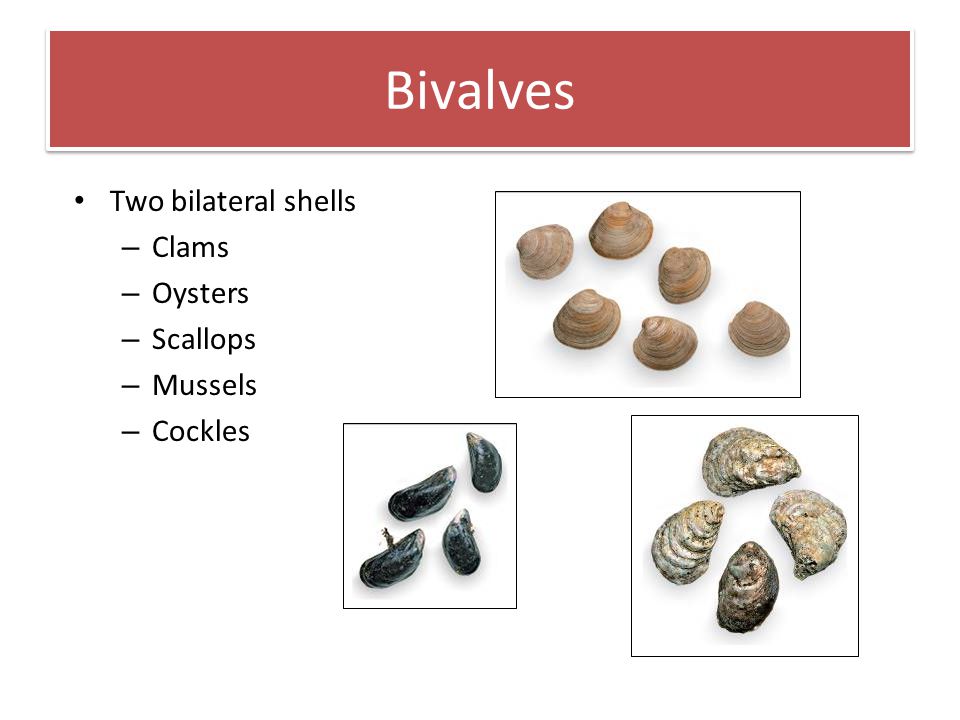The image serves as an informational template on bivalves, prominently featuring the word "Bivalves" in white text situated on a red rectangular background with a white border at the top. Below this header, there is a bulleted list that describes bivalves as organisms with "two bilateral shells," followed by a sub-list of examples: clams, oysters, scallops, mussels, and cockles. To the right of this text, the image includes three separate groups of bivalves, each set within black rectangular borders. The topmost group contains about six brown-shelled objects, likely clams. The middle group consists of four black-shelled objects, possibly mussels. The bottom group displays four grayish-brown objects, potentially other types of bivalves. The image visually conveys the variety and characteristics of bivalves through detailed text and corresponding photographs.